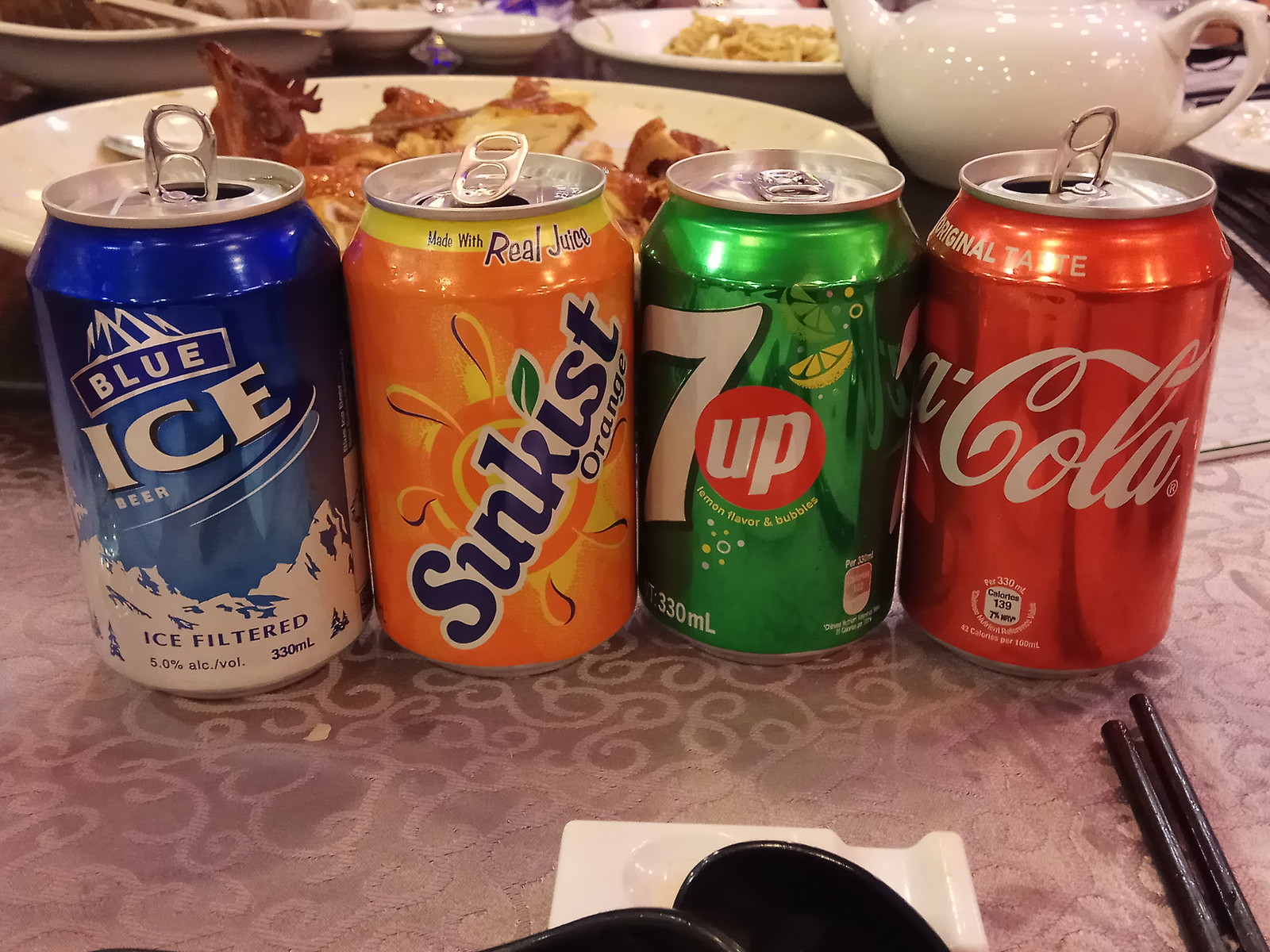This photograph captures a bustling restaurant scene, centered around a light gray table with a mahogany edge. Prominently displayed are four beverage cans arranged left to right: a blue ice beer can adorned with snowy mountain silhouettes, an orange Sunkist soda, an old-style green 7-Up can with a red dot, and a classic red Coca-Cola can. Among these, only the 7-Up remains unopened. The table, set against a pink tablecloth, also holds a pair of black chopsticks at the bottom right, suggesting an Asian dining influence. Scattered white plates with remnants of a meal, which includes items like French toast, sausage, and scrambled eggs, fill the background. A white ceramic teapot sits to the upper right, adding a touch of elegance to the lively and cluttered scene.